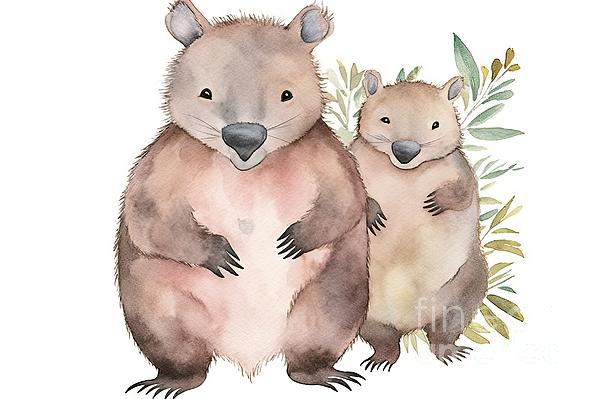A whimsical watercolor illustration features two rotund, cartoon-style woodland creatures resembling mother and baby bears. Both bears are depicted standing with arms positioned curiously over their chests. The larger bear on the left, with brown fur accented by a cream-colored belly, has a prominent black nose, small black eyes, and visible whiskers, along with black-tipped paws and feet. The smaller bear to the right mirrors the larger bear's appearance, emphasizing the familial bond with identical fur coloration and features. Surrounding the baby bear, an array of colorful foliage composed of greens, browns, yellows, and some bluish-pink accents creates a vivid backdrop. This charming image, set against a stark white background, has a subtle watermark in the lower right corner that reads "FIN." The style and composition suggest an illustration intended for a children's book, highlighting the anthropomorphic and endearing nature of the bear duo.